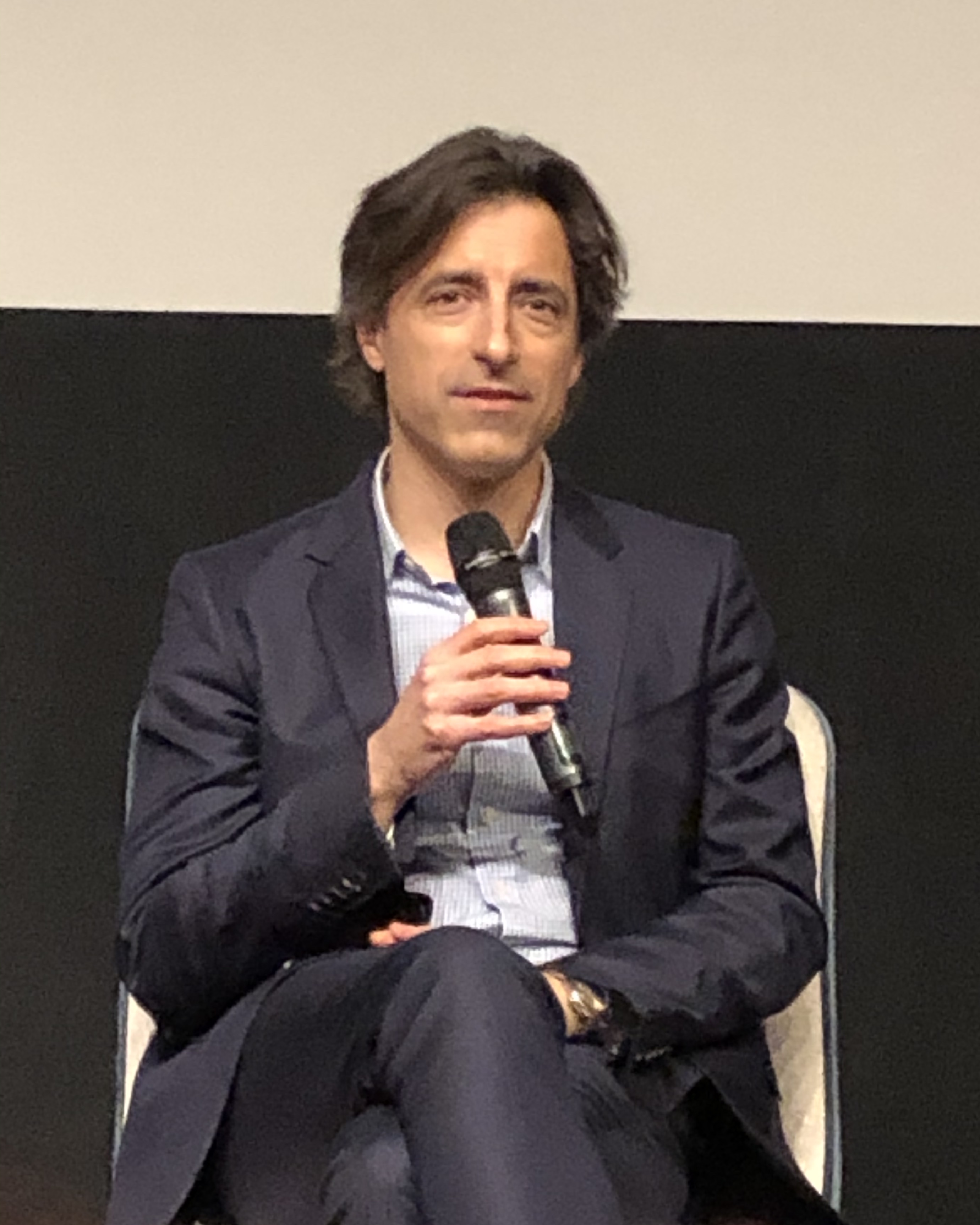The image captures a man seated in a chair, appearing to be in the midst of an interview. His right hand firmly grasps a black microphone, indicating he's preparing to speak while attentively listening. The man has wavy brown hair that reaches the nape of his neck and brown eyes. He is dressed in a black suit jacket and pants, paired with a blue and white vertically striped collared shirt that is unbuttoned at the top. His left wrist sports a luxury gold watch. The chair he sits on has a tan cushion with gray trim. The background wall is black up to his ears, transitioning to a beige or tan color above his head. He sits with one hand in his lap, legs crossed, and looks towards the center-left of the image.